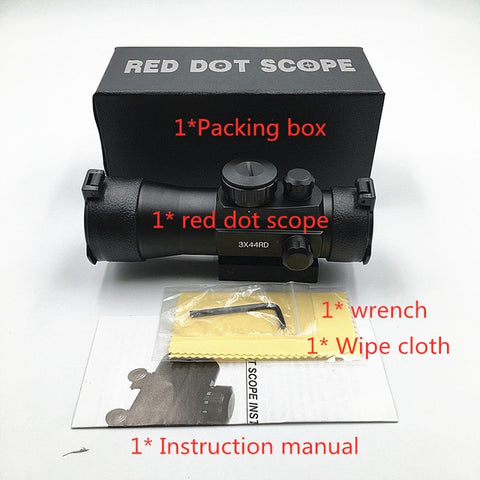This image showcases the complete packaging contents of a rifle-mounted scope product. At the back is a black box prominently labeled in gray text with "Red Dot Scope," featuring a crosshair in the center of the "O." This box is also marked with red text indicating "1x Packing Box." In front of the box, the black scope itself is visible, engraved with "3X44RD" and labeled "1x Red Dot Scope" in red text. The scope has adjustment dials on its side and top, as well as protective caps on both ends. 

In front of the scope lies a white piece of paper, identified as the "1x Instruction Manual." On top of this manual is a small plastic bag containing an Allen wrench and a yellow microfiber cloth, with red text labeling the items as "1x Wrench" and "1x White Cloth." This setup clearly details all the components included in the purchase of this red dot scope package.